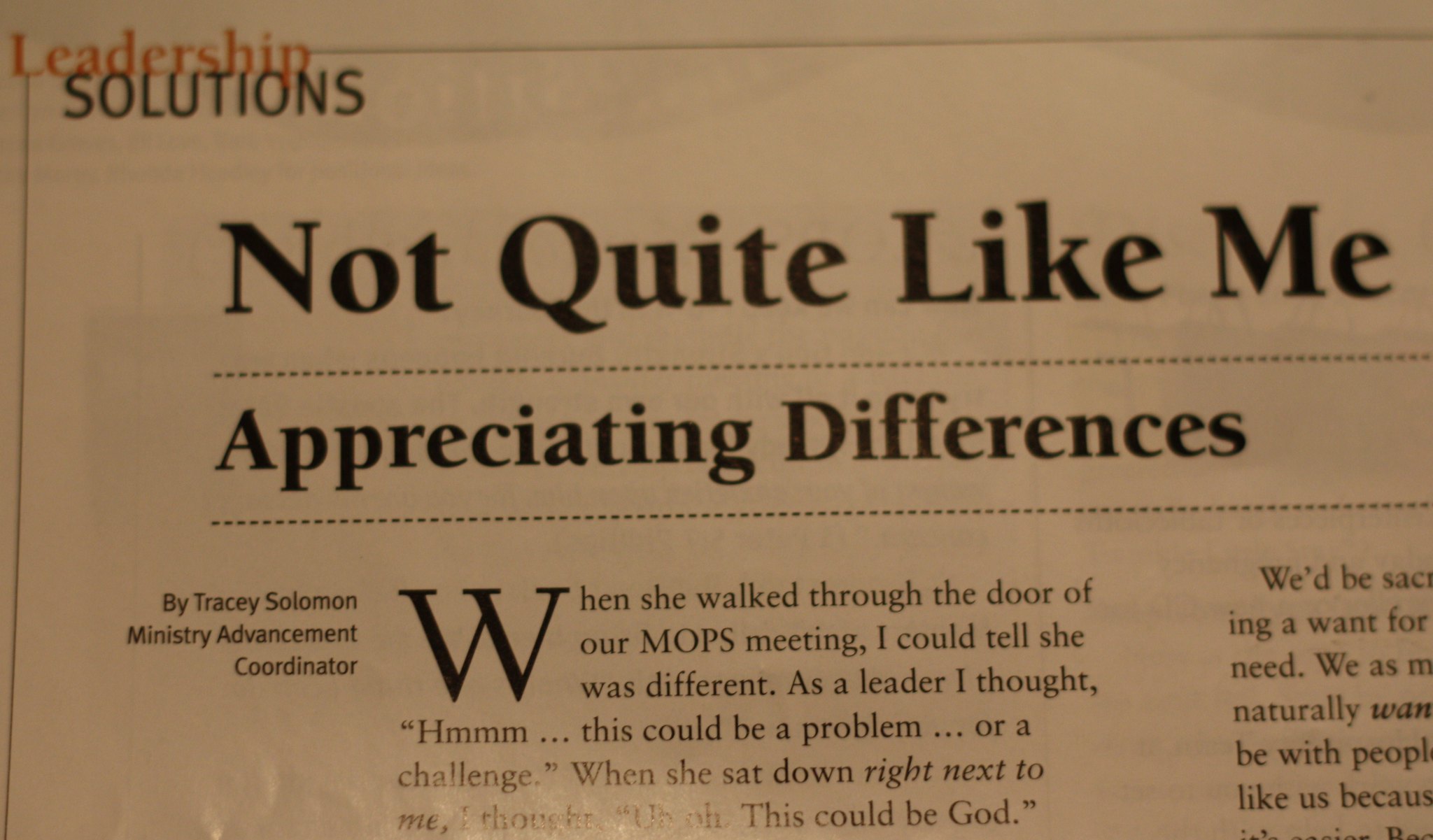This image captures a glossy page from a magazine or newspaper. The paper appears aged with a beige or dark brown hue. In the top left corner, the publication's title, "Leadership Solutions," is displayed, with “Leadership” in red and "Solutions" in black capital letters. The article's bold title, "Not Quite Like Me," is followed by a byline, "Appreciating Differences." The article is authored by Tracy Solomon, labelled as the Ministry Advancement Coordinator. The first paragraph starts with a prominently large and bold 'W,' reading: "When she walked through the door of our MOPS meeting, I could tell she was different. As a leader, I thought, hmm, this could be a problem or a challenge. When she sat down next to me, I thought, uh-oh, this could be God." The image only partially captures the page, cutting off a secondary column of text to the right.